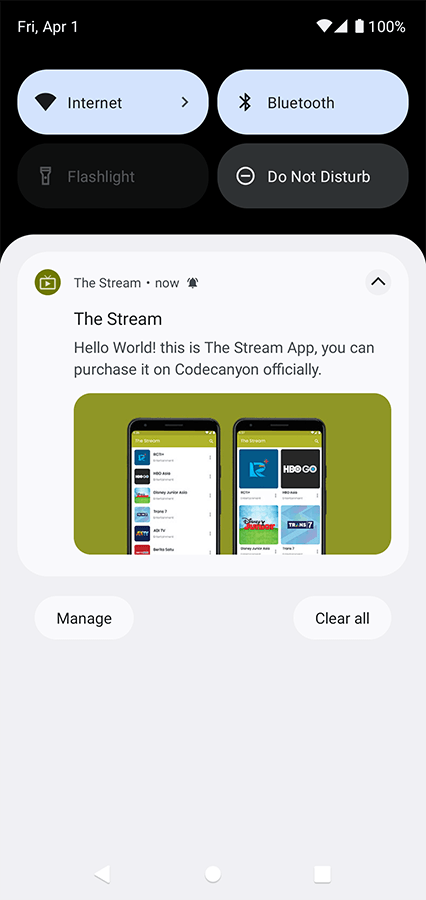The image appears to be a screenshot taken from a smartphone, showcasing its notification and quick settings panel. 

At the top, the status bar displays the date and time as "Friday, April 1st," alongside icons for Wi-Fi connectivity, cellular signal strength, and a fully charged battery at 100%. 

Below the status bar, there are four quick setting buttons. The two blue ones are for "Internet" on the left and "Bluetooth" on the right, while the two black buttons below them are labeled "Flashlight" and "Do Not Disturb."

The central part of the screenshot features a white notification panel displaying a message from an app called "The Stream." The message reads, "Hello world. This is a stream app. You can purchase it on CodeCanyon officially." The notification background is green within a horizontally elongated rectangle. 

The notification shows two black cell phones with different layouts. The phone on the left has six images with text on a white background, though the text isn't clearly legible. The phone on the right displays a grid of four larger images, arranged in two rows, partially cut off at the bottom.

At the bottom of the notification panel, there are buttons labeled "Manage" and "Clear All," likely for managing and dismissing notifications, respectively.

Finally, the bottom part of the screenshot shows the phone's navigation bar with three icons: a backward arrow for navigating back, a circle for returning to the home screen, and a square for viewing recent apps.